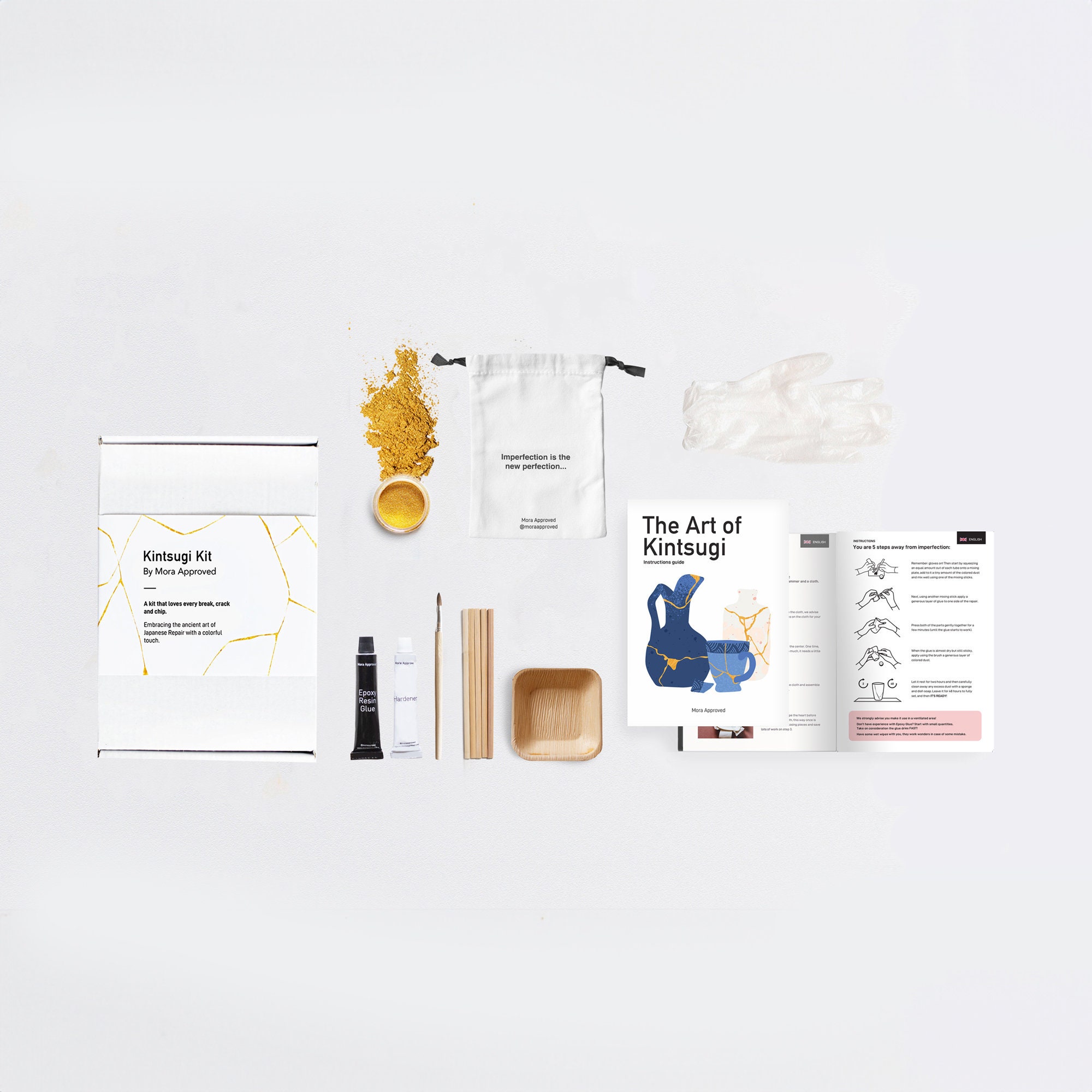The image depicts an advertising display of a comprehensive Kintsugi Kit by Mora Approved, set against a pristine white background. The kit contains eleven distinct items meticulously arranged for viewing. On the left, a white box boldly labeled "Kintsugi Kit by Mora Approved" introduces the set. Accompanying it are two small tubes, one clearly marked as "Epoxy Resin Glue" and the other, which is unreadable, likely also containing a bonding agent. A paintbrush with a pine-colored handle stands beside four wooden sticks resembling chopsticks. Below, a shallow, square wooden bowl sits next to a circular container filled with shimmering gold powder, some of which is artfully spread around the container. Adjacent to these, a white fabric bag with dual black drawstrings is elegantly inscribed with "Imperfection is the new perfection..." Above the bag, a pair of clear plastic gloves is included for handling materials, and a booklet titled "The Art of Kintsugi" provides instructions. This curated collection embodies the spirit of Kintsugi, offering a poetic embrace of flaws through meticulous repair.